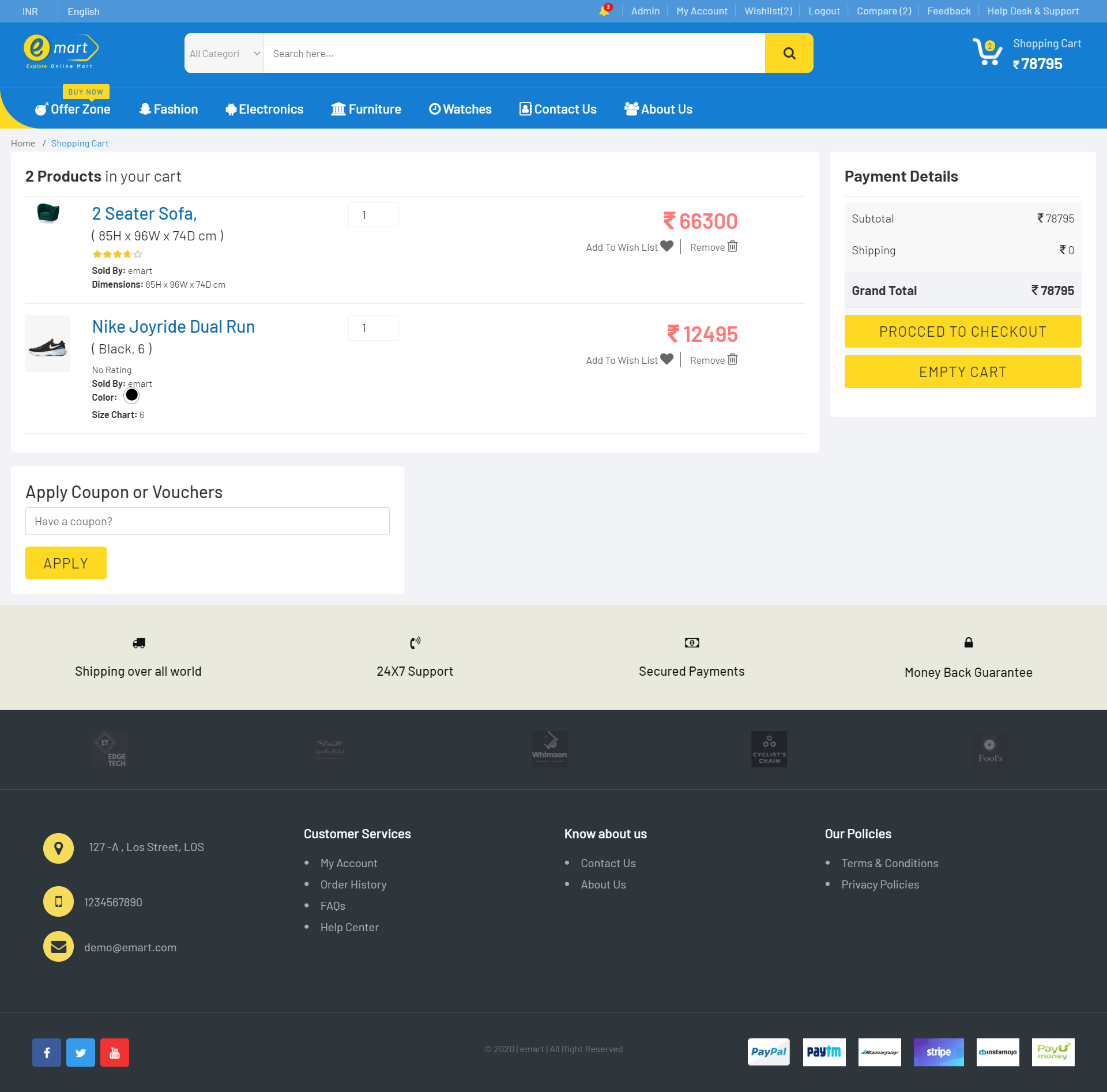This screenshot captures an e-commerce website displaying a shopping cart summary. At the top of the page, there is a blue rectangular header, giving the website a distinct, organized look. The cart contains two items: a two-seater sofa priced at 66,300 (currency unspecified), and a pair of Nike Joyride Dual Run size 6 black shoes priced at 12,495 (currency unspecified). Each item in the cart has options to add it to a wish list or remove it, indicated by a trash can icon.

The interface also features several functional buttons highlighted in yellow, such as a magnifying glass icon for search, and two prominent buttons to "Proceed to Checkout" and "Empty Cart." Additionally, there is a section titled "Apply Coupon or Vouchers," marked by a clickable yellow box, which enhances user convenience by allowing them to benefit from discounts.